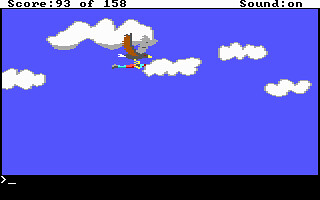In this captivating image, a computer game scene is portrayed. At the top of the display, the text "Score: 93 of 158" is prominently featured in black characters against a white background. Next to it, the words "Sound On" are also clearly visible.

The majority of the screen is filled with a darkish shade of blue, reminiscent of a twilight sky. Scattered across this blue expanse are five clouds, each with irregular, squiggly shapes. These clouds are predominantly white with gray edges, giving them a slightly ominous appearance.

Centrally positioned between two of the clouds is a figure that captures the viewers' attention. This figure appears to be a person wearing gray and black shoes, blue pants, and a red top. Perched on or hovering above this individual is a creature with light brown and light gray wings. It seems to be either landing on or falling towards the person, adding an element of dynamic action to the scene.

At the very bottom of the screen, there is a solid black bar, possibly indicating a user interface element or a ground line, grounding the animated suspension in the sky above. This detailed caption helps to vividly describe the intriguing scenario presented in the image.